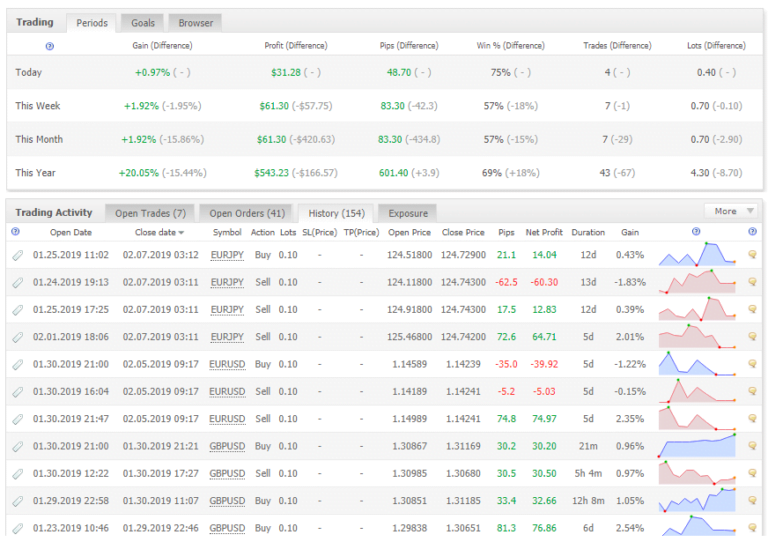**Descriptive Caption:**

The image depicts a detailed trading dashboard featuring two prominent sections. At the top, there is a larger box with a smaller gray and white striped box nested within it. The top row of the primary box is labeled "Trading" and includes three tabs titled "Periods," "Goals," and "Browser." Beside these tabs, a blue circle with a black question mark serves as a help icon. Below this, a white stripe lists various metrics: "Gain Difference," "Profit Difference," "Pips Difference," "Win Percent Difference," "Trades Difference," and "Lots Difference." The performance indicators show positive results for today, this week, this month, and this year, highlighted in green. The specific differences for trade volumes stand at four, seven, seven, and forty-three, followed by the lots difference.

The second large box also features gray and white stripes. At the top, it is labeled "Trading Activity" and includes various tabs: "Open Trade (7)," "Open Orders (41)," "History (154)," "Exposure," and an additional drop-down menu for more options. Another blue circle icon, likely indicating more information, is beside these tabs. This section details trading specifics such as open date, closed date, symbol, action, lots, SL price, TP price, open price, closed price, pips, net profit, duration, and gain. On the right-hand side of this section, a graph visually represents the sales data.